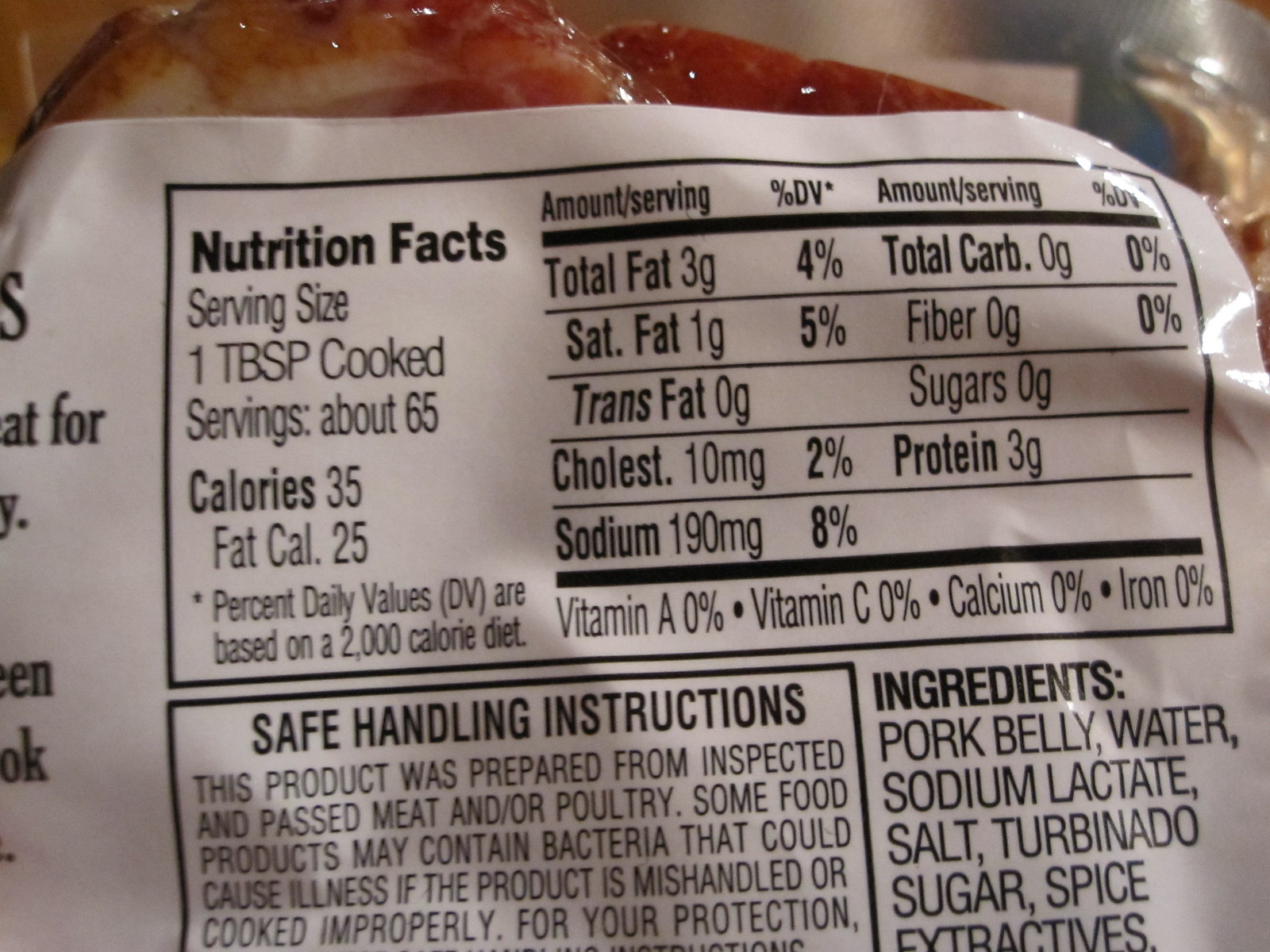This image shows a transparent package of meat, likely pork belly or honey baked ham, with a grayish background and visible pink meat marbled with fat. The packaging contains a white nutrition label detailing that the serving size is one tablespoon of cooked meat, with approximately 65 servings per package. Each serving provides 35 calories, of which 25 are from fat, and includes 3 grams of protein. The nutritional breakdown also highlights 4% total fat, 5% saturated fat, 2% cholesterol, and 8% sodium, with no carbohydrates or sugars. Despite the presence of turbinado sugar in the ingredients, the sugar content per serving is negligible. The ingredients listed are pork belly, water, sodium lactate, salt, turbinado sugar, and spice extractives. The label also includes safe handling instructions, indicating that the meat was inspected and passed, and cautioning about potential bacteria if mishandled or improperly cooked.